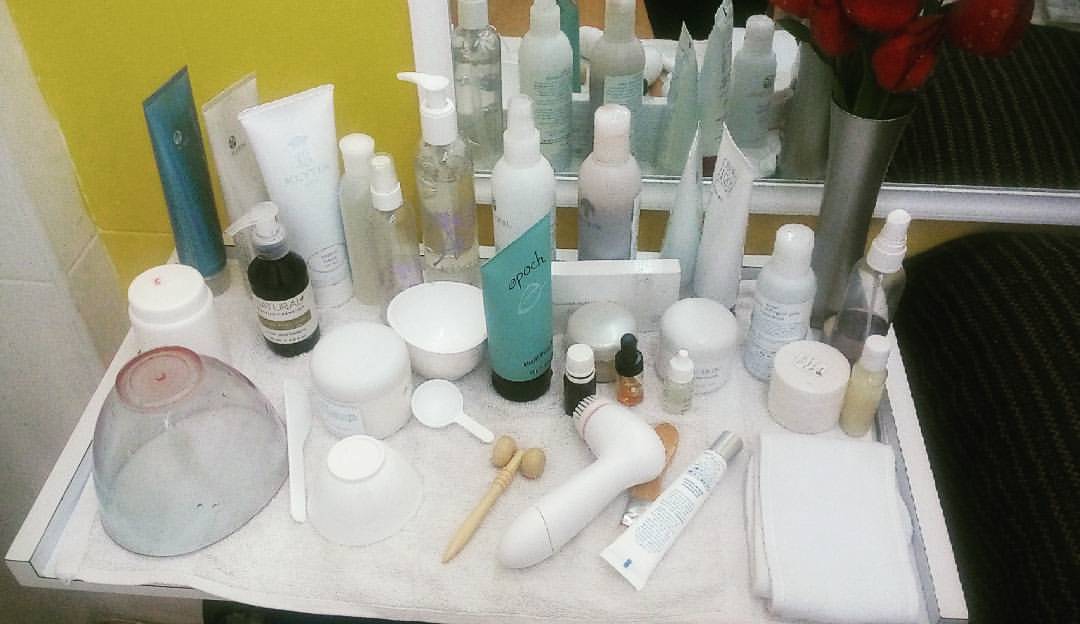This overhead photograph captures the surface of a cabinet, possibly located in a bathroom or at a bedside. The backdrop features a yellow wall transitioning into a white corner on the left. A white-framed mirror stands prominently on the right side, reflecting part of the scene. A quilted brown coverlet or sofa back is visible in the far right background.

On the cabinet's surface, a neatly folded white towel serves as a base for various personal hygiene items. In the right corner, a tall, cylindrical silver bud vase with a flared top showcases a bouquet of vibrant red roses. Beside the vase, an upside-down transparent glass bowl with a slightly pink base sits atop the towel. Scattered around are several tubes of personal hygiene products and a plastic white face scrubber, its brush end facing towards the left, adding to the practical yet homely arrangement.